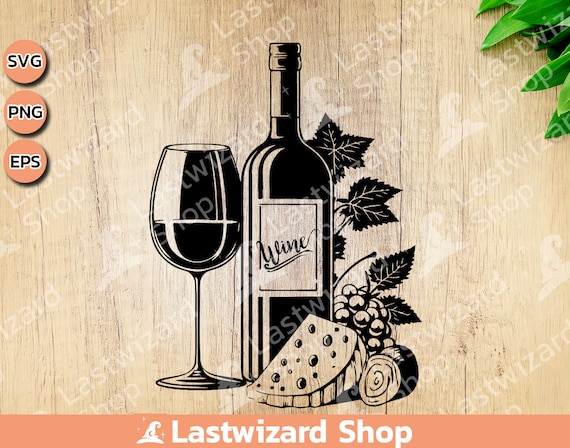The image is an advertisement for the Last Wizard Shop, prominently showcasing a bottle of wine, a glass of wine, cheese, grapes, and grape leaves. The background is designed to resemble wood, with the text "Last Wizard Shop" repeatedly faded in white across it. The advertisement’s elements are mostly in black and white, with the text "Last Wizard Shop" in white at the bottom. Central to the image are the wine bottle, the half-full wine glass, and the cheese. There are three small peach-colored circles in the upper left corner labeled SVG, PNG, and EPS, while green leaves add a splash of color in the upper right. The image also features a peach-colored border at the bottom.